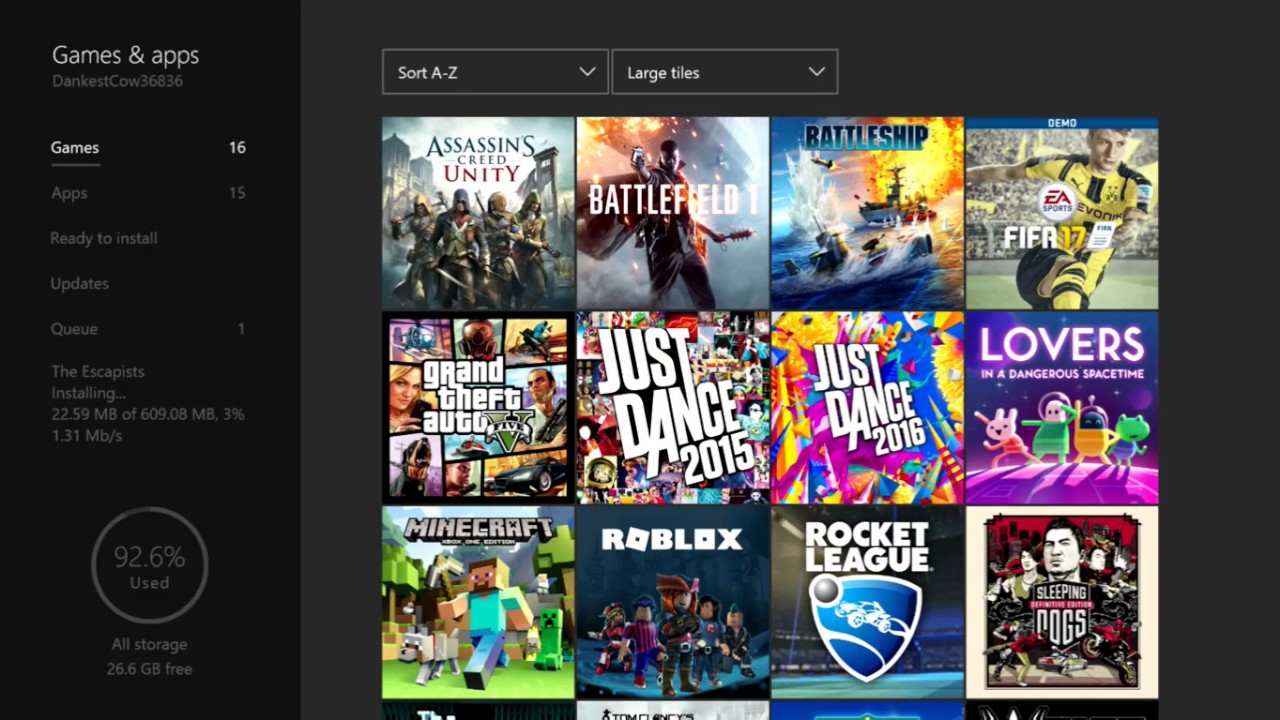The image depicts a digital interface showcasing a person's game and app collection. In the upper left-hand corner, the header reads "Games and Apps." Below the header is a list displaying multiple numeric values: "Darkest or Dankest Cow, 36, 8, 36", indicating game statistics or IDs. Underneath, a categorization summary notes "Games: 16," "Apps: 15," and tabs titled "Ready to Install," "Updates," and "Queue."

Highlighted prominently is an installation progress bar for the game "Escapists," which shows 22.59 MB of 609.08 MB downloaded, reflecting a 3% completion rate at a speed of 1.31 MB/s. Additionally, the interface indicates that 92.6% of storage is used, leaving 26.6 GB free.

Centered on the screen is a drop-down menu for sorting options labeled "Sort A to Z" alongside another for display settings named "Large Tiles." The visible part of the user’s collection includes titles such as "Assassin's Creed Unity," "Battlefield 1," "Battleship," "FIFA 17," "Grand Theft Auto V," "Just Dance 2015," "Just Dance 2016," "Lovers in a Dangerous Spacetime," "Minecraft," "Roblox," "Rocket League," and "Sleeping Dogs."